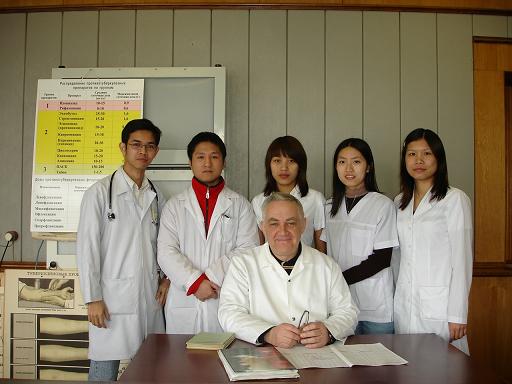The indoor photo captures a detailed scene within what appears to be a medical or educational setting. Centered at a wooden table with a light gray, wooden slat wall and a dark brown ceiling, an older white man in a white lab coat is seated, holding a pair of glasses. In front of him are three books and some papers. Behind him, standing in a line and looking at the camera, are five people, seemingly students of Asian descent, also wearing white lab coats. Among them are three women and two men, with the man on the left wearing a stethoscope. The setting includes a brown wooden door to the right and a television mounted on the wall behind them which has a white, pink, and yellow poster attached, with other posters underneath. While the older man and one woman are smiling, the rest appear neutral or sullen.